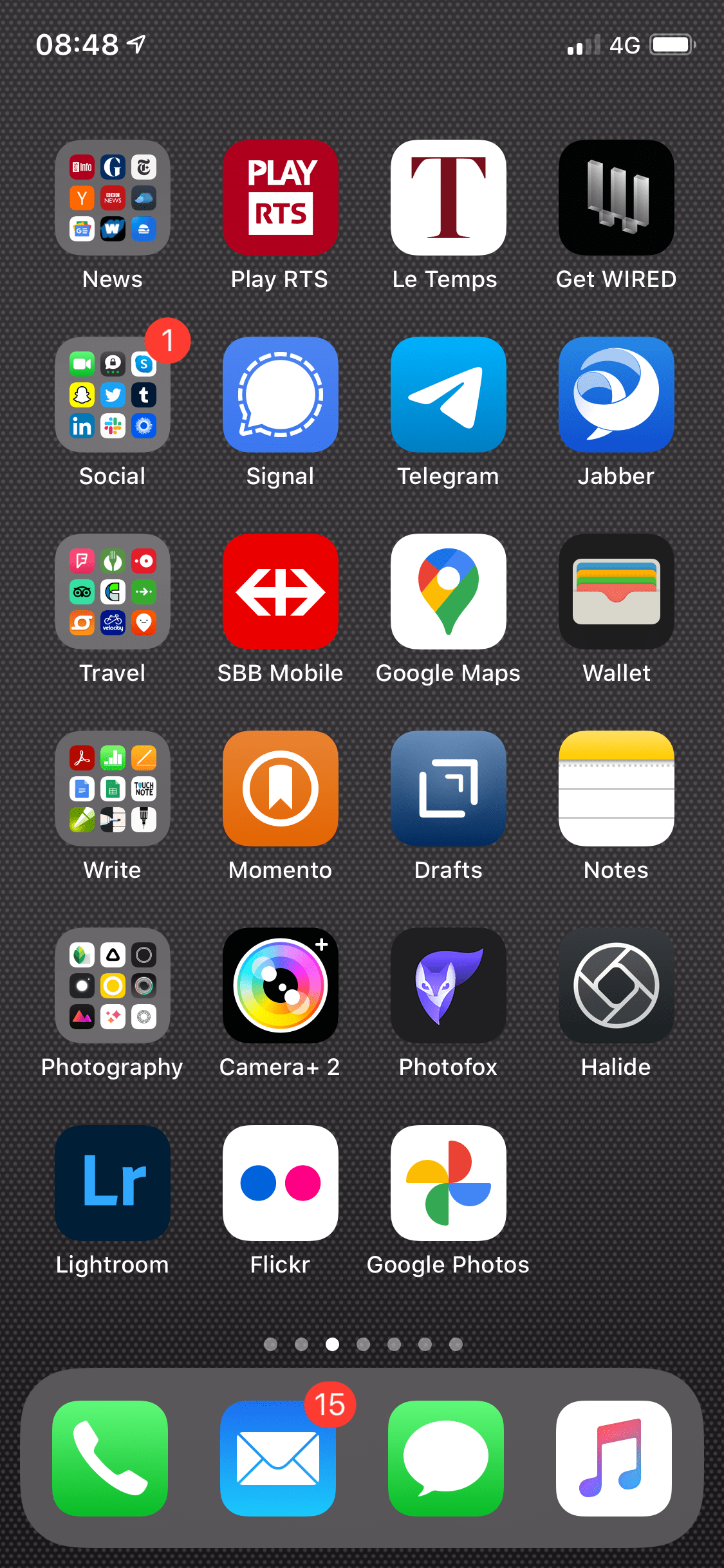This screenshot captures the detailed appearance of a mobile phone's home screen. The background features a mesh-like texture that resembles a gray canvas. Positioned at the top left corner in white font, the time is displayed as 8:48, accompanied by a location sharing icon indicating that location services are active.

On the upper right side, the mobile signal strength is shown as two out of four bars, with the "4G" symbol next to it. A fully charged battery icon is also present, depicted in white.

Beneath these indicators, the home screen is organized into a grid of app icons and folders, arranged in rows of four. Here's a detailed breakdown:

**Top Row:**
1. **Folder labeled "News"** - Contains six apps related to news.
2. **Play RTS** - An app likely for media or games.
3. **Attempts** - The purpose is unclear but could be task-related.
4. **Get Wired** - Possibly a tech or news app.

**Second Row:**
1. **Folder labeled "Social"** - Filled with various social media apps.
2. **Signal** - A secure messaging app.
3. **Telegram** - Another messaging platform.
4. **Jabber** - Yet another app for messaging.

**Third Row:**
1. **Folder labeled "Travel"** - Houses apps useful for traveling.
2. **SMB Mobile** - Purpose is unclear but could be business-related.
3. **Google Maps** - Navigation and maps app.
4. **Wallet** - Likely a digital wallet for payments.

**Fourth Row:**
1. **Folder labeled "Right"** - Contains unspecified apps.
2. **Memento** - Possibly a reminder or notes app.
3. **Drafts** - Likely for document or note editing.
4. **Notes** - Standard note-taking app.

This structured layout allows the user to quickly access their most-used apps and folders efficiently.